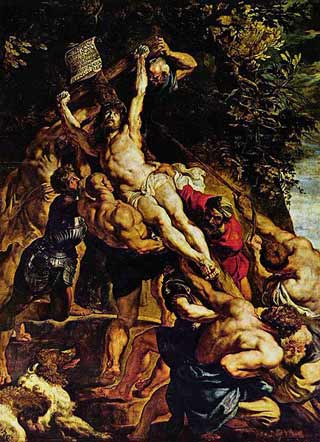This detailed painting, known as "Elevation to the Cross," captures the dramatic moment of the crucifixion with a dark and somber atmosphere. Central to the image is a muscular, nearly nude Jesus, shrouded only by a loincloth, his hands and feet nailed to a cross. The cross is shown tilted to the right, being hoisted by several muscular figures, their upper bodies bare and straining as they position it into the ground. A man in a red coat holds Jesus' hip and lower leg, seemingly aiding in the elevation process, while another figure, donned in what appears to be a metallic uniform, assists below. 

In the background, a mix of foliage and dark, ominous sky adds to the painting's intense mood. A large tree with green and yellowing leaves towers over the scene, its presence almost overshadowing the tragic event. To the right of the composition, subtle hints of water can be seen. Additionally, a brown and white dog with its tongue out is positioned at the bottom left corner, adding a curious yet poignant detail to the tableau. The entire scene is dense with action and emotion, capturing the gravity of the crucifixion through its dark tones and crowded biblical figures.